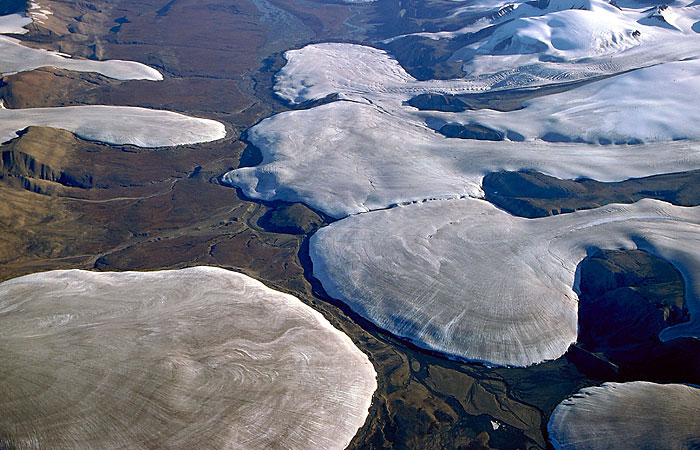The image, taken from a high vantage point that could be mistaken for a satellite view, captures a striking landscape during the daytime. It showcases a dry, brown land area interspersed with large patches of what appears to be white and light gray snow or ice. The snow forms circular shapes that flow into the rocky terrain, suggesting either melting ice pulling back or streams bringing the snow down. Predominantly, the upper right corner of the image is filled with white and light cream-colored glaciers, which have dirty brown hues near their meeting points with the ground. The glaciers appear smooth, with no sharp edges, indicating slight movement or melting. The darker brown landmasses are visibly interspersed among these glaciers, with horizontal lines marking certain areas at the bottom. The overall scene is a blend of stark white, light gray, and various shades of brown, creating a contrasting yet cohesive depiction of this unique landscape.